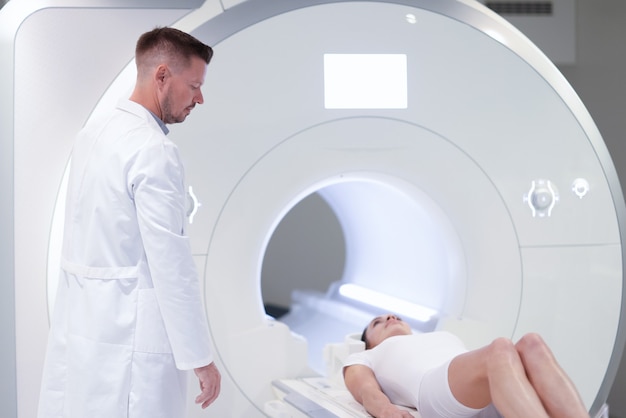In this detailed photograph, a female patient wearing an all-white outfit is positioned on a sliding table of an MRI machine. The table, partially retracted into the large circular opening of the machine, underscores the room's clinical ambiance. The MRI machine dominates the image, characterized by its expansive, light and dark gray rounded casing, and illuminated from within by fluorescent lights. A white rectangular panel at the top middle of the machine further enhances this illumination. The patient lies supine with her knees slightly elevated, her head rested comfortably on a cushion, and her arms resting at her sides, extending off the image at the ankles. To the left, a doctor with short black hair, possibly a beard, and wearing a long white lab coat attentively monitors the patient, ensuring her alignment. His brown hair contrasts with the sterile white setting, and his posture reflects a careful and professional demeanor as he overlooks the patient’s preparation for the scan. The office setting is minimally featured, with hints of a vent located in the top right corner, emphasizing the clinical and controlled environment where this medical procedure unfolds.